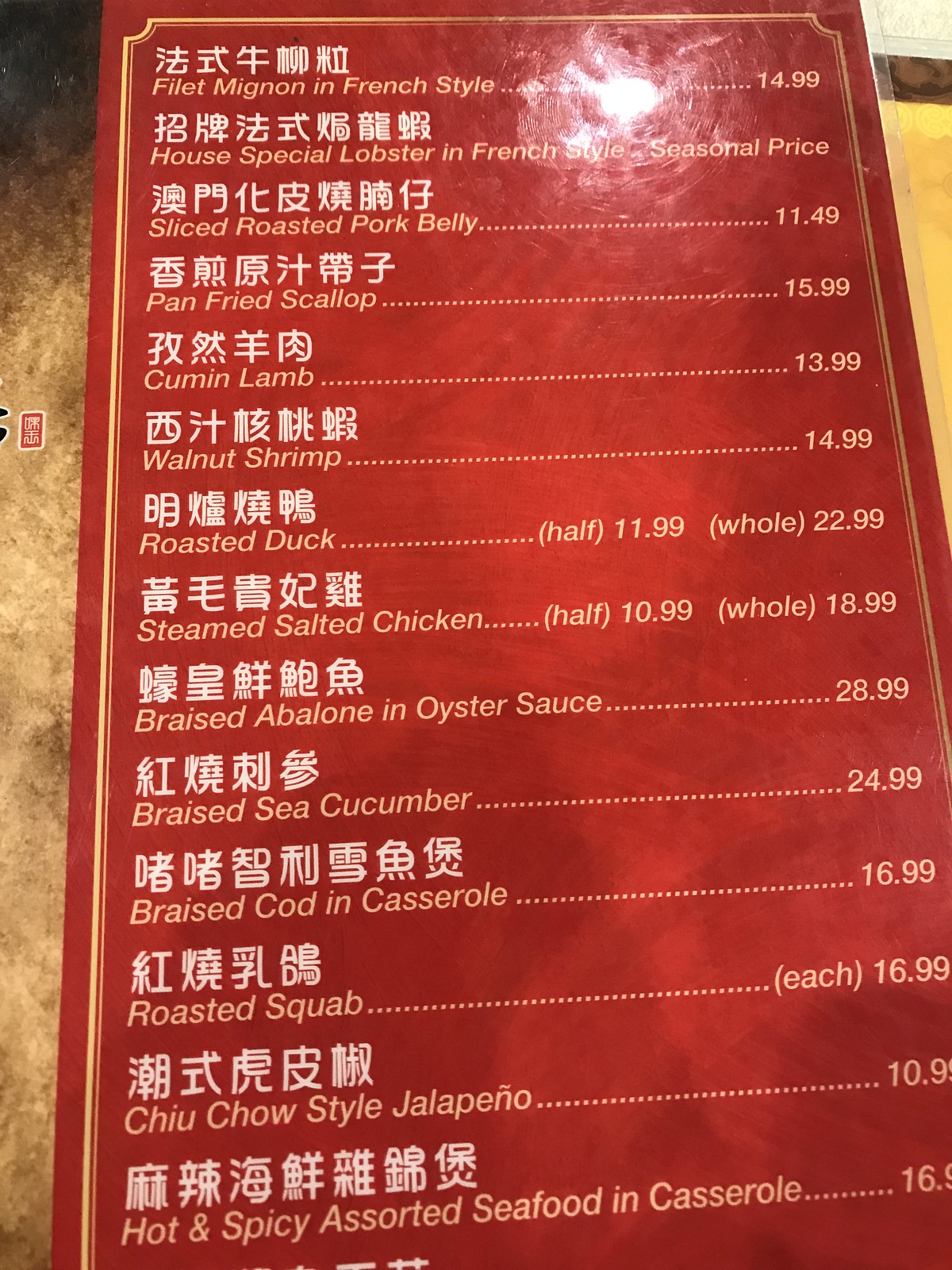A rectangular photograph of a restaurant menu, with the longer sides forming the left and right edges, showcases only a portion of the menu due to its partial framing. The menu dominates the left side of the image and appears slightly tilted, with the bottom part of the menu appearing larger due to the angled perspective. The visible section of the menu has a red background, adorned with peach-colored English text listing various food items and their prices. Above the English descriptions, there are corresponding dish names written in white Asian characters. The dishes listed are as follows: 

1. Filet Mignon in French Style - $14.99
2. House Special Lobster in French Style - Seasonal Price
3. Slice Roasted Pork Belly - $11.49
4. Pan Fried Scallop - $15.99
5. Cumin Lamb - $13.99
6. Walnut Shrimp - $14.99
7. Roasted Duck - Half: $11.99, Whole: $22.99
8. Steamed Salted Chicken - Half: $10.99, Whole: $18.99

The menu, though partially visible, offers a glimpse into the diverse culinary offerings of the restaurant, punctuated by both familiar and specialty dishes, each paired with a price to entice potential diners.